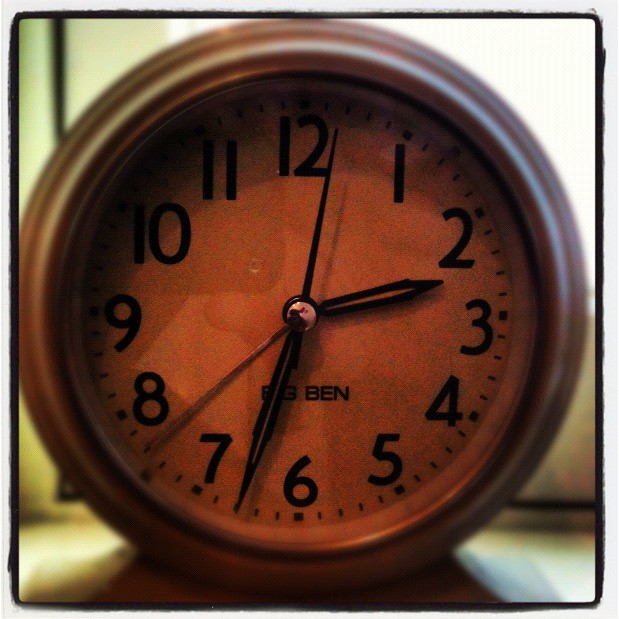This photograph features a vintage circular clock with a distinctively aged aesthetic. The clock face, characterized by an orangish-brown to light brown hue, prominently displays black numerals from 1 to 12, with 12 positioned at the top and 6 at the bottom. Surrounding the numerals are small black lines indicating each minute. The clock features three black hands and one long, slender silver hand. At its center, where the hands converge, there is a silver metal circle overlaying a black circle. Positioned beneath the clock’s hands is the text "Big Ben" in black lettering. The clock frame, crafted from a silvery-gray metal, is slightly blurred, as is the background, which draws complete focus to the detailed and intricate face of the clock.